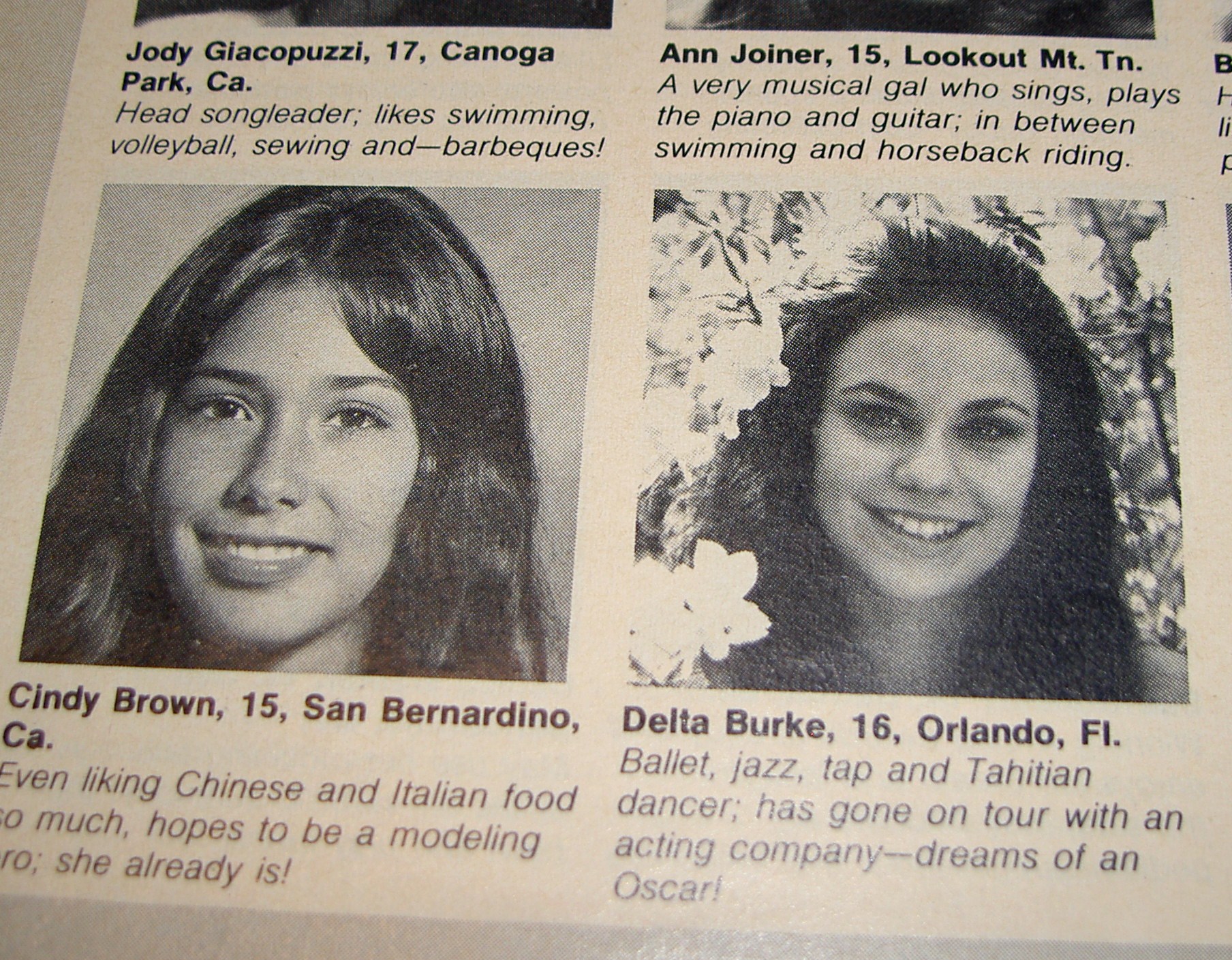This black-and-white photograph resembles a yearbook page featuring four captioned portraits of young women. The leftmost section displays Cindy Brown, a 15-year-old from San Bernardino, California, with long dark hair, described as someone who enjoys Chinese and Italian food and dreams of becoming a model, a career she is already pursuing. Beside her is Delta Burke, a 16-year-old from Orlando, Florida, with long dark hair, highlighted as a ballet, jazz, tap, and Tahitian dancer who has toured with an acting company and aspires to win an Oscar. The top sections include Jody Giancarlozzi, a 17-year-old from Canoga Park, California, identified as the head song leader who enjoys swimming, volleyball, sewing, and barbecues; and Ann Joyner, a 15-year-old from Lookout Mountain, Tennessee, portrayed as a musical gal who sings, and plays the piano and guitar, alongside engaging in swimming and horseback riding. The photograph captures Cindy in a straightforward headshot while Delta’s image is set outdoors among flowers.